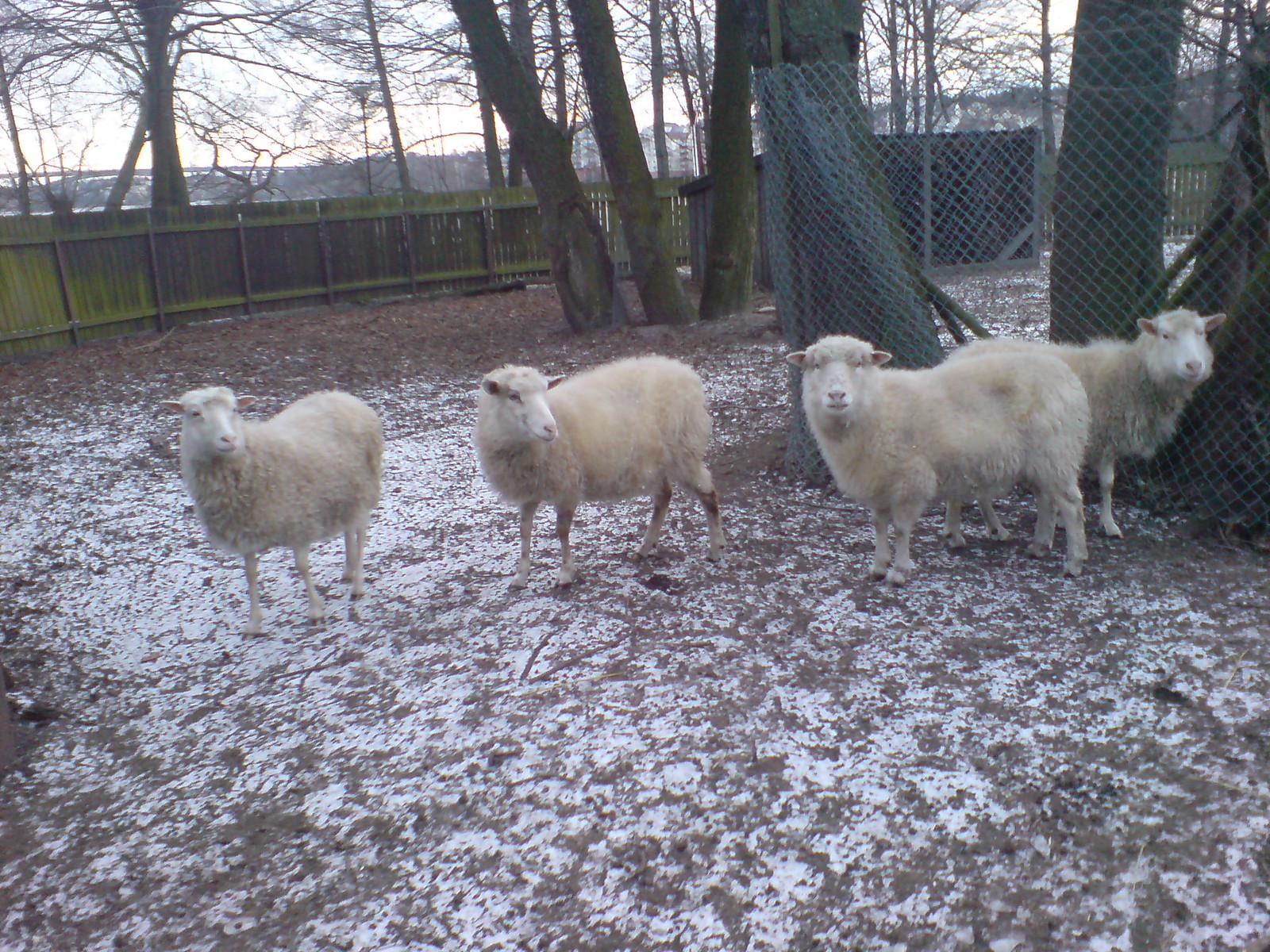The photograph captures a serene winter scene in a large backyard or enclosed pen. The ground is covered lightly with snow, revealing patches of dirt beneath. Among the barren trees that rise sporadically from the yard, a wooden fence, marred with mold and algae, wraps around the area, providing a rustic boundary. In the background, particularly in the top right corner, a wooden structure resembling a barn is partially visible, suggesting a shelter for the animals.

The focal point of the image is four sheep, positioned prominently near the foreground. These adult sheep, mostly white with hints of gray and beige, possess thick but well-maintained coats, suggesting they are prepared for the cold. Two of the sheep gaze directly into the camera, while the other two look off to the right, adding a dynamic feel to the otherwise quiet setting. Beyond the fence, trees devoid of leaves stand against a gray sky, adding to the wintry and somber atmosphere. The distance reveals an escarpment or a rise, suggesting landscape variations on the far side of a nearby river or terrain. The sheep, standing on their skinny legs with ears protruding sideways and a slight pink tinge, add a charming contrast to the otherwise dreary day.